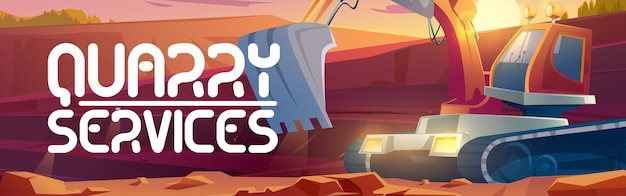This image features a thin, rectangular banner depicting a computer-generated, cartoon-style illustration of an orange excavator amidst a quarry setting. The excavator, with its metallic housing and sizable gray bucket, is positioned prominently in the rocky foreground, supported by its black treads. Its cabin, which has a blue glass window and two illuminated lights, stands out against the backdrop. The quarry walls behind it are colored in rich tones of red and brown, while the sunset sky peeks over the rugged terrain. On the left-hand side, white text in a digital font reads "Big White Texas' Quarry Services." The overall scene is imbued with the warm hues of the setting sun, highlighting the detailed and vibrant environment.